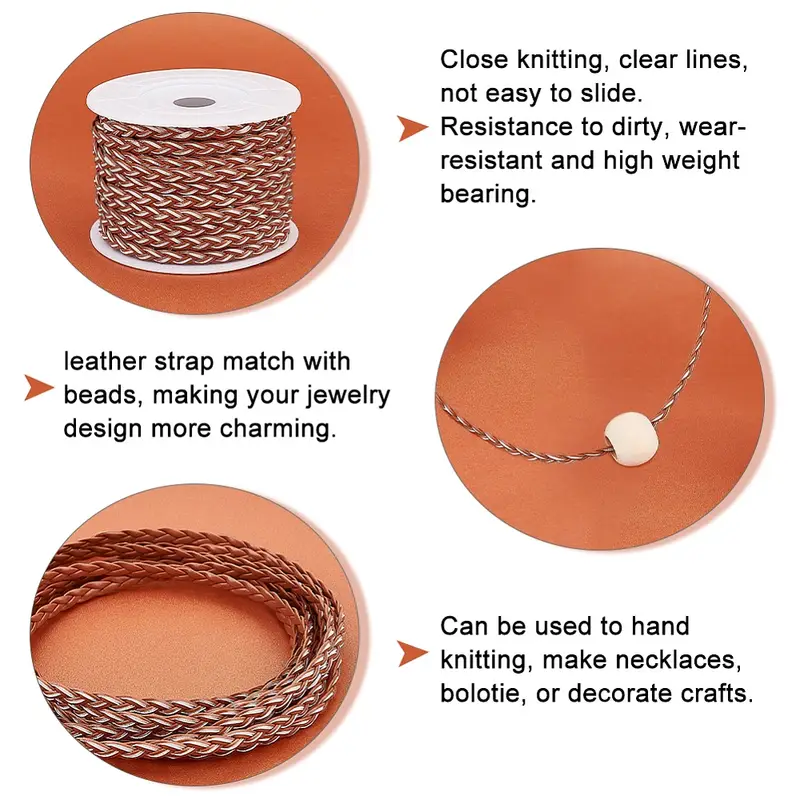The image showcases a detailed promotional diagram of a durable and versatile leather knitting material, with a tan, beige backdrop. Divided into three sections, each featuring a circular photograph with an orange background, the image provides in-depth information about the product's features and applications. In the top section, a white plastic spindle wrapped with brown and white braided leather strips is depicted, accompanied by text that highlights its close knitting, clear lines, resistance to dirt, wear resistance, and high weight-bearing capacity. The middle section displays a white bead threaded onto the braided leather, elucidating how the leather strap can match with beads to create charming jewelry designs. Lastly, the bottom section shows the coiled leather strips and explains that the material can be hand-knitted to make necklaces, bolo ties, or decorated crafts, making it a versatile crafting item. All the text is written in black, providing clear and essential details about the product's characteristics.